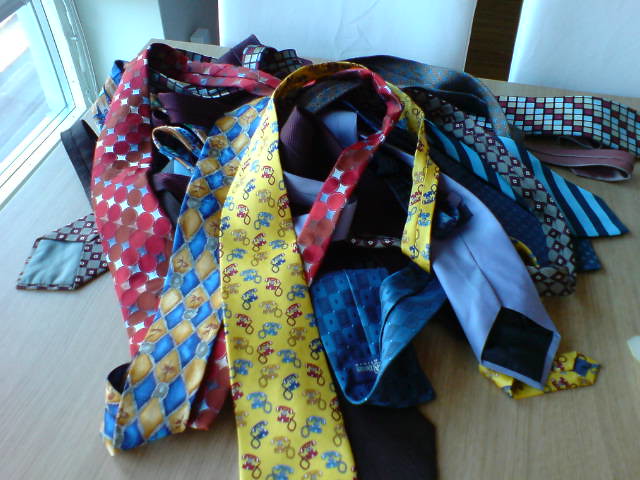The photograph captures a chaotic pile of approximately 20-30 neckties, spread haphazardly across a light wooden table. The ties exhibit a vibrant array of colors and designs, including a notable yellow tie adorned with tiny telephone-like shapes, another featuring a gold, brown, and blue diamond pattern, and others with intricate tile or geometric patterns. There are solid colored ties as well, such as a deep blue and a purple one. This colorful assortment of ties sits in what appears to be an office-like room; a window on the left side allows daylight to illuminate the scene. Behind the table, three paper-like boxes with small openings are visible, alongside what appears to be a plug. The background also reveals a white wall and darker shadows, adding depth to the overall setting.